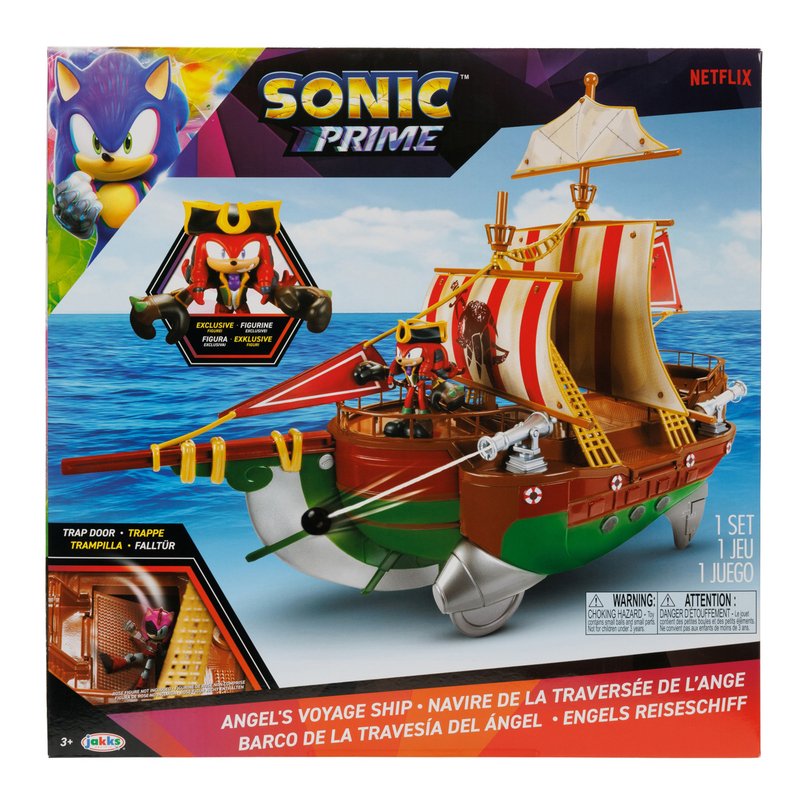The image showcases the detailed box art of a Sonic the Hedgehog-themed pirate ship toy from the Sonic Prime TV show. In the top left corner, a cartoon image of Sonic the Hedgehog is prominently displayed. The top edges feature a black border containing the Sonic Prime logo, with a Netflix logo in the top right corner. The central focus of the artwork is a green and brown pirate ship with wood-like plastic textures, white sails adorned with red stripes, wood banisters, and yellow netting on the sides. Knuckles the Echidna stands at the bow of the ship, donning a black and yellow pirate hat and black gloves. The ship is equipped with silver cannons, one of which is shown firing a cannonball attached by a string. In the bottom left corner of the box, text says "Trap Door" next to an image of Amy Rose falling through a trap door. The bottom features a red border with white multilingual text that reads "Angel's Voyage Ship," "Navier de la Traverse de la Ange," "Barco de la Traversia del Angel," and "Angel's Raceship." A small square warning label, including a choking hazard warning in English and French, is located above the text in the bottom right corner. The entire package is targeted for ages 3 and up, as indicated by the logo in the far bottom corner.